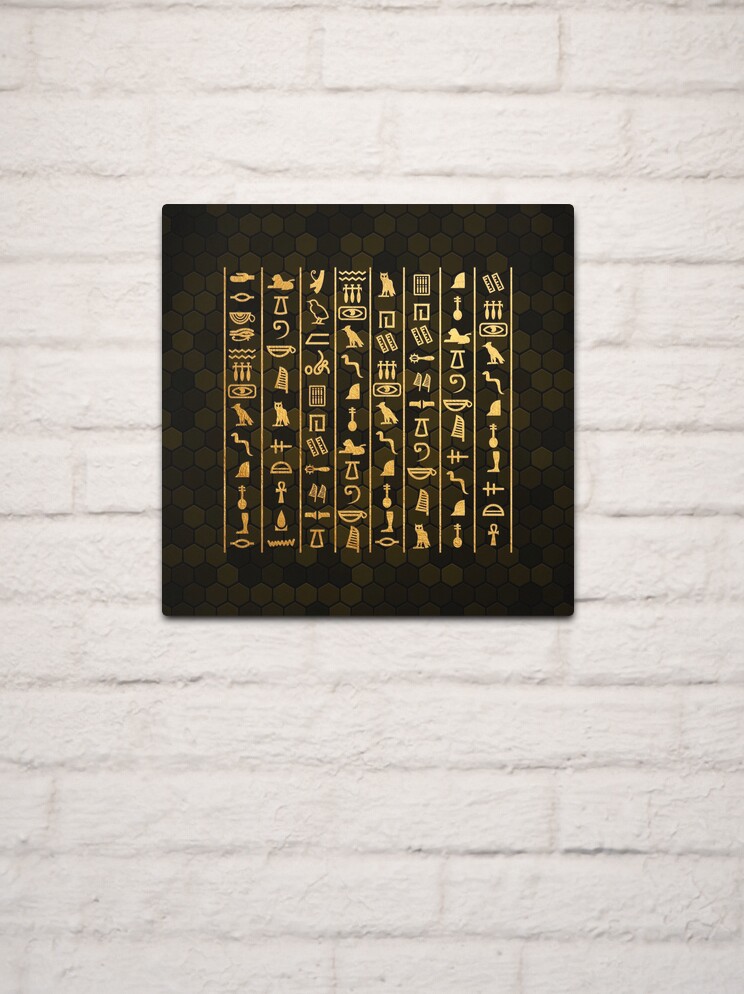The image showcases a piece of art hanging prominently on a white brick wall, characterized by smaller, uniform bricks. The photograph's background wall is slightly muted and out of focus, drawing attention to the centrally placed artwork. This piece features a thick black border and an interior background that appears black or dark green. The artwork itself is divided into eight to nine vertical columns, filled with numerous ancient or hieroglyphic-like symbols, arranged in rows varying from 10 to 12 items each. These symbols, rendered in gold or yellow, are reminiscent of ancient signage. The art is mounted against the brick wall, covering the area equivalent to about six sets of bricks, and emanates a light that creates no shadows, enhancing its detailed and intricate presentation.